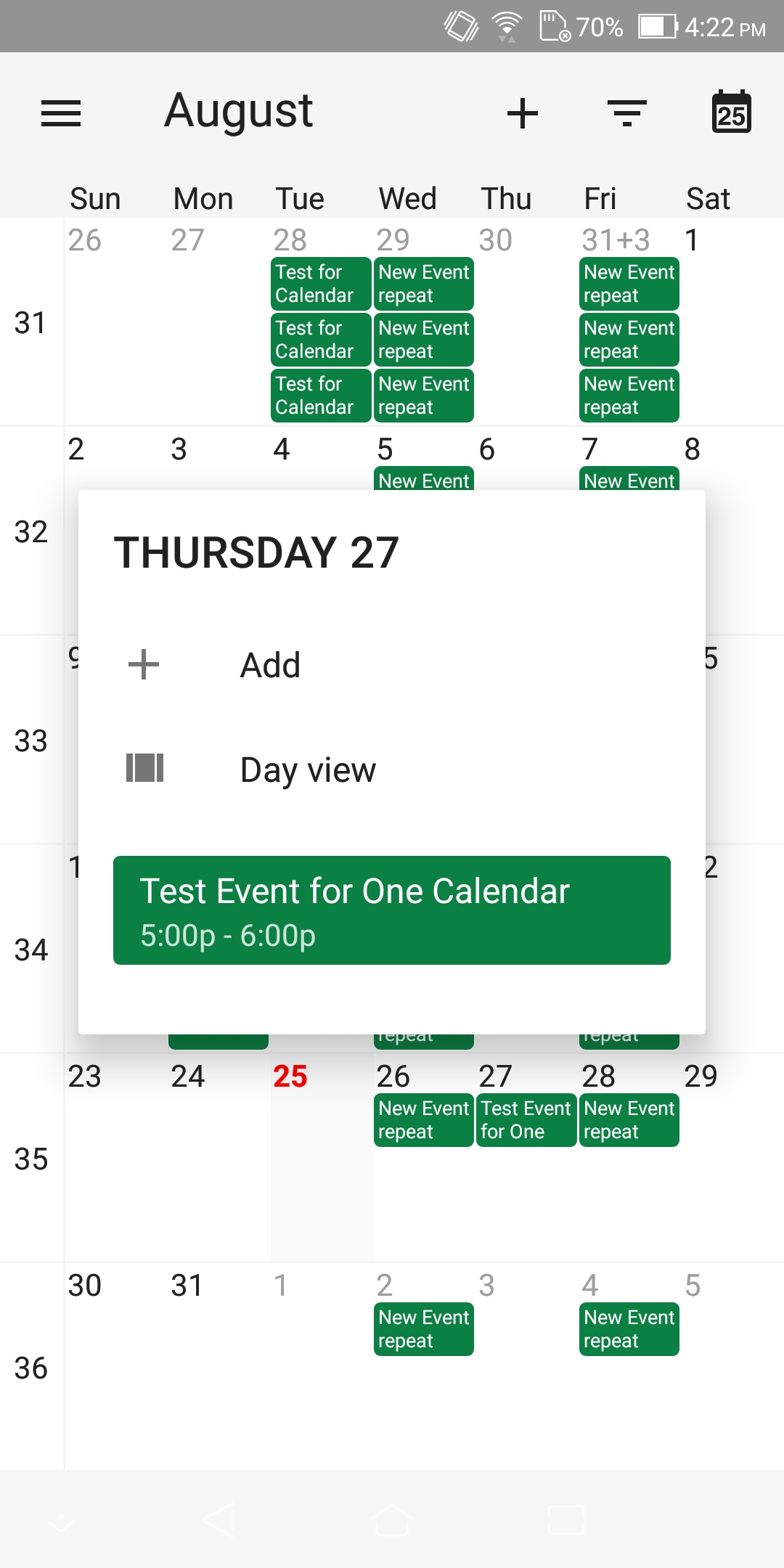The image showcases a detailed view of a digital calendar interface, likely resembling Google Calendar, set to August 25th (year unspecified). The calendar's clean design features a predominantly white background with black numerals marking each date. Upon selecting a date, the numeral turns red and the date's background shifts to light gray, highlighting the chosen day.

In this image, a user appears to be testing the calendar's functionalities. Various test events have been added, labeled with names like "test for calendar" and "new event repeat." The user’s current focus is on August 27th, where a specific event titled "test event for one calendar" is scheduled from 5 PM to 6 PM. Additional features such as 'add buttons' and a 'day view' option are also visible, providing the user with further interaction capabilities and calendar management options.